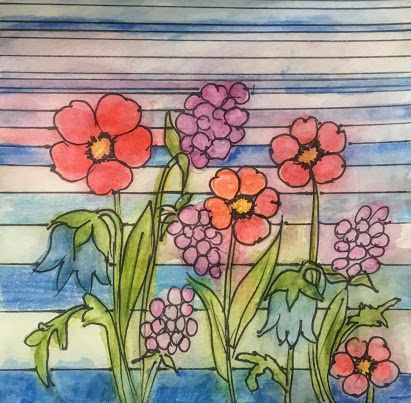This image is a detailed watercolor drawing with a blue and white striped background, accented by light pinks and purples. The flowers, outlined in black, are prominently featured in the foreground. Each flower has five petals with a yellow center surrounded by black fibers, all attached to green stems with leaves. The composition includes several different flowers: four round flowers with a central yellow spot and black details, a blue upside-down flower, and a purple flower that might resemble a lilac or a hyacinth. The artist used thin black lines to define the petals and flower shapes, with additional elements like buds, leaves, and stems meticulously colored in green. The background stripes give a sense of a lightly patterned wall, contributing to the overall aesthetic nature of the drawing.